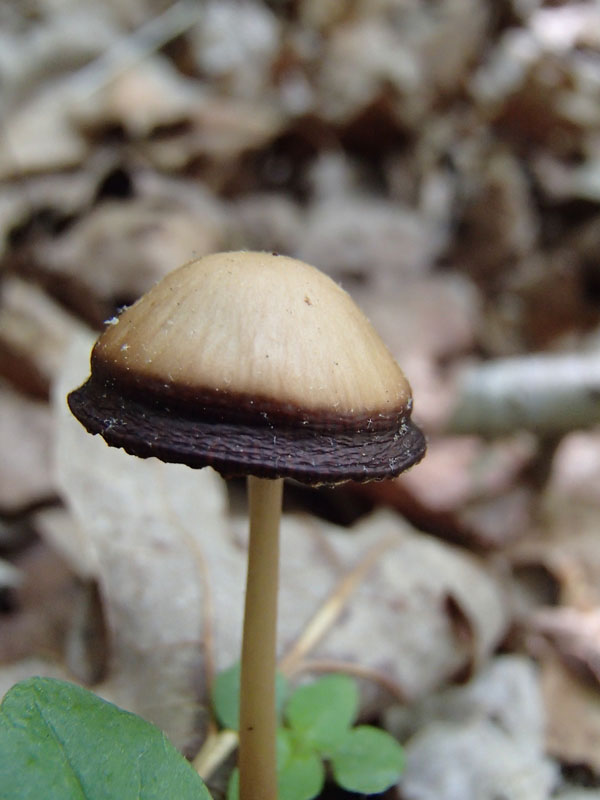The image captures a close-up of a wild mushroom growing amidst a mix of green clover and brown, dead leaves, suggesting a moist environment. The mushroom features a rounded, tan cap with a brownish base and a light beige stem. The scene hints at a fall time setting, evidenced by the presence of dead leaves and brown tones in the background, which is slightly blurred. Additionally, some white specks, perhaps pollen or dirt, are noticeable on the mushroom's surface. Other details include green leaves in the bottom left corner and the surrounding earthy setting with bits of dirt and possibly other small elements like stones and worms. The overall setting indicates a vibrant, natural habitat for the mushroom.